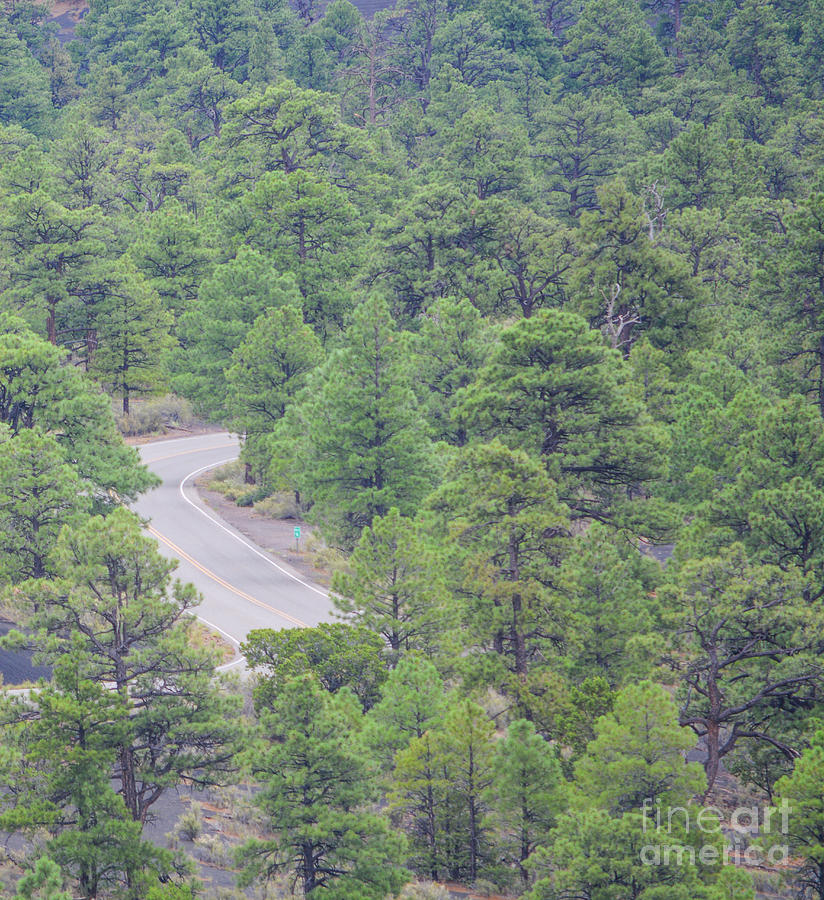This image features a captivating aerial view of a dense forest dominated by various shades of green from different species of trees, including many pine trees and others in yellowish-green hues. The forest is intersected by a two-lane highway that curves to the right. This road is marked with a yellow no-passing stripe in the center and solid white lines on either side. Alongside the highway, brown dirt areas and bushes are visible, adding texture to the scene. In the upper-right section of the image, there appears to be a green sign with white writing, though its details are not fully discernible. The scene is devoid of cars, accentuating the natural beauty of the forest landscape. The photograph bears the watermark "Fine Art America" in gray text in the lower right corner, indicating its origin from a company specializing in nature scenes.